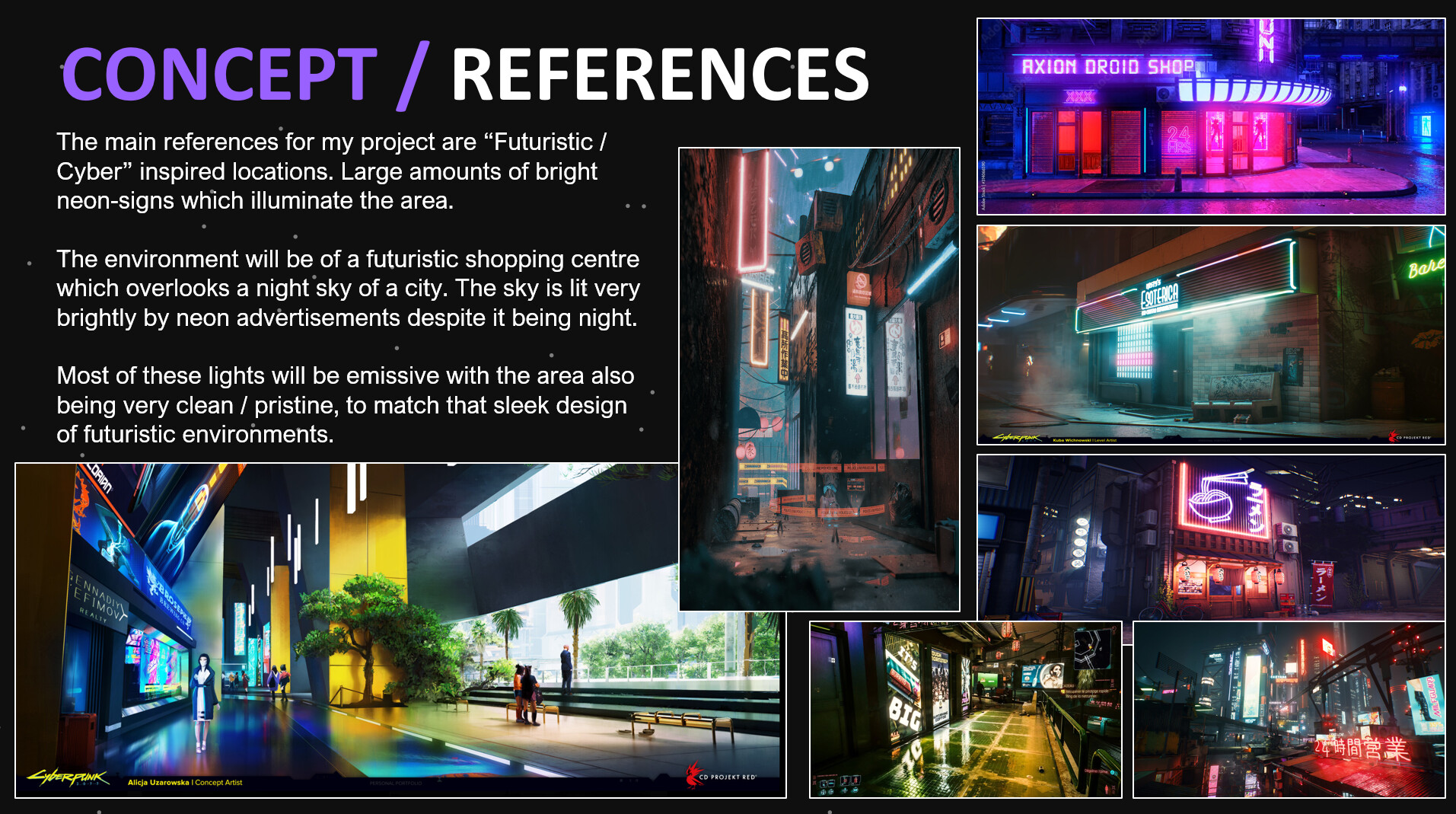This striking image is a landscape-oriented collage featuring seven vibrant photographs that capture futuristic, neon-lit environments. Dominating the top left corner in purple and white capital letters, the text reads "CONCEPT / REFERENCES." Below this, smaller white text provides a detailed explanation: "The main references for my project are futuristic/cyber-inspired locations. Large amounts of bright neon signs illuminate the area. The environment will be a futuristic shopping center that overlooks a city night sky, aglow with neon advertisements. These lights are largely emissive, contributing to a clean and pristine atmosphere that epitomizes sleek futuristic design."

The collage includes a variety of photographs in both vertical and horizontal orientations. Prominently featured are exterior views of buildings adorned with an array of neon lights and signage, conjuring images of bustling, high-tech urban centers. One notable photograph in the top corner showcases a brilliantly lit building, while another at the bottom presents a modern office interior, bathed in neon light. The overall backdrop is a deep black, highlighting the luminous colors and intricate lighting, effectively blending photographic realism with graphic design aesthetics. The composition elicits a vivid sense of a futuristic metropolis bathed in surreal, colorful glow.